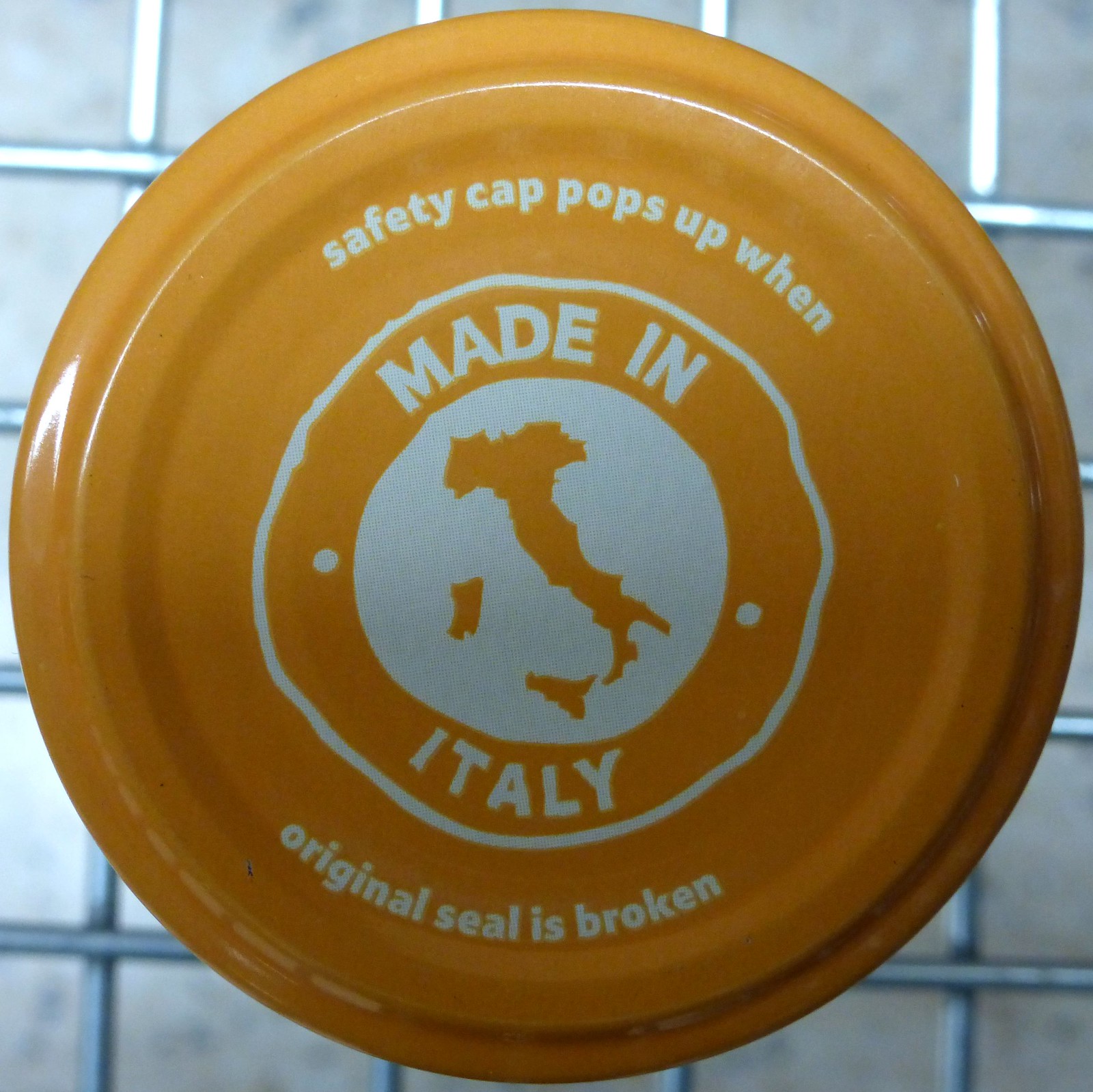The image depicts a large, round orange safety cap, likely the top of a jar, with white lettering. The cap prominently displays the text "Safety cap pops up when original seal is broken." In the center of the cap, there is a jagged white circle featuring a map of Italy. Below the map, the cap reads "Made in Italy," flanked by white dots on either side. The background reveals the item sitting in a shopping cart, with a silver metal grate and a whitish-gray tiled floor visible through the cart's grid. The lighting is poor, with a slight highlight in the upper left corner, but the details on the cap remain discernible.